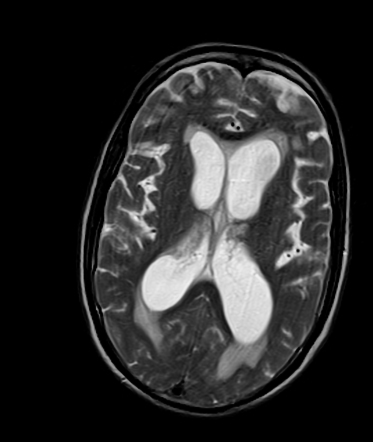The image is a black and white MRI scan depicting a cross-section of a human brain placed against a large, square, black background. In the center of the image, an oblong, oval shape represents the skull, slightly tilted to the right. Inside this oval, intricate details of the brain are clearly visible. The brain's creases and crevices are predominantly white, running vertically from the top center to the bottom center of the image. The scan captures various structures within the brain, including some large, white, circular formations nestled within the brain's creases. The brain's front is oriented towards the top of the photo, with the back positioned at the bottom. The white matter outlined within the brain creates an almost X-like pattern at the center of the image, enhancing the visual detail of the brain's internal structure. The image lacks any text, allowing the detailed anatomy of the brain to be the focal point.